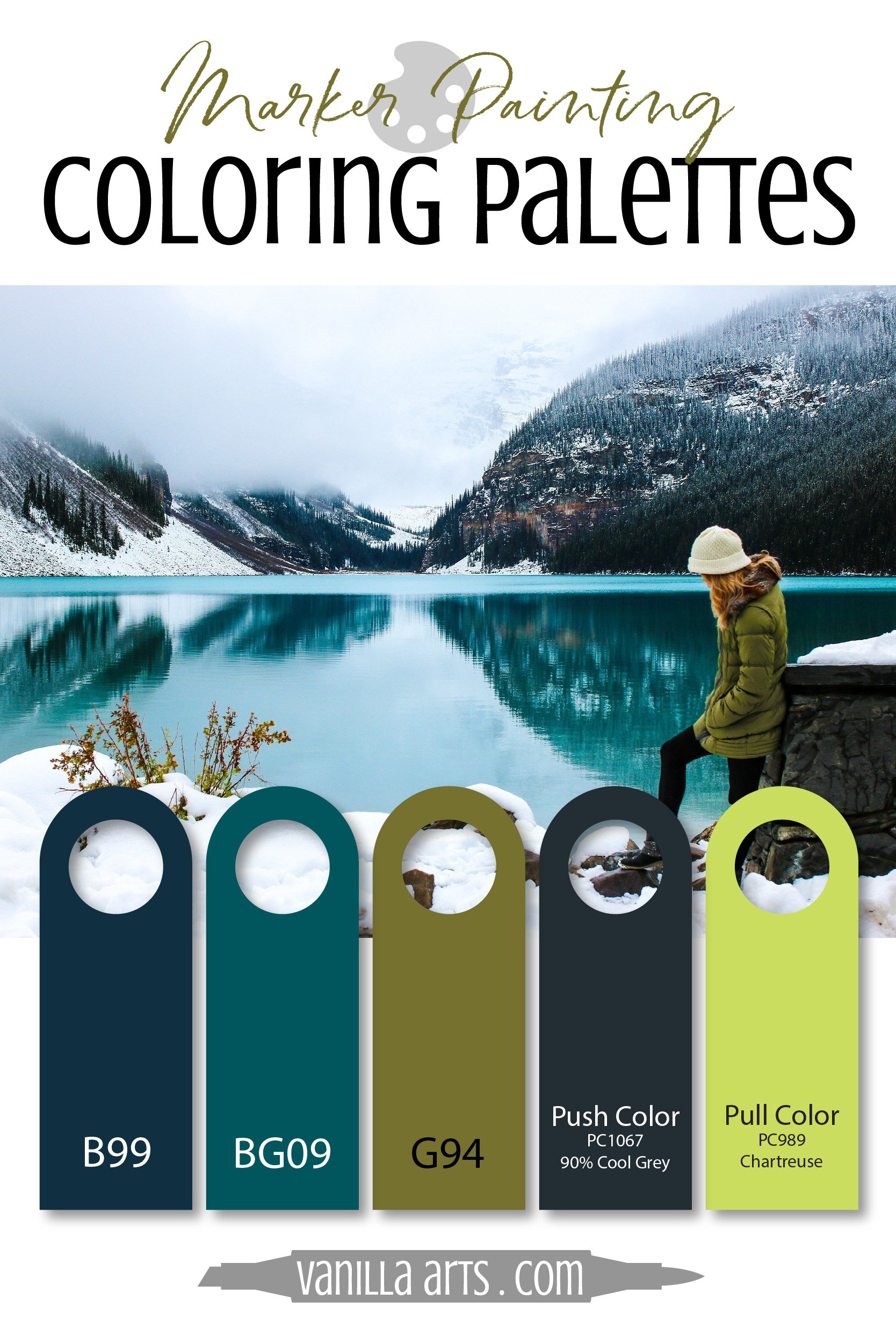This vertical banner graphic features an advertisement set against a white background with a serene winter scene. At the top, the green cursive text reads "Marker Painting" with a gray painter’s palette icon nestled between the words. Below, large black letters spell out "Coloring Palettes." The centerpiece of the ad is a photo of a woman with light brown hair standing on snow-covered ground, overlooking a tranquil, reflective blue lake. The lake is surrounded by fog-shrouded, mountainous hills adorned with evergreen trees. The woman, positioned on the right side of the image and leaning against a pillar, is dressed in a white knitted beanie, an olive-colored green jacket, and black tight pants with boots. Along the bottom of the image are five color swatches drawn from the visual elements in the photo: the first swatch is labeled B99 in dark blue, the second is BG09 in teal, the third is G94 in olive, the fourth is PC1067 90% Cool Gray in dark grayish blue, and the fifth is PC989 Chartreuse in a yellowish green. At the very bottom of the poster, the URL "vanillaarts.com" is prominently displayed.